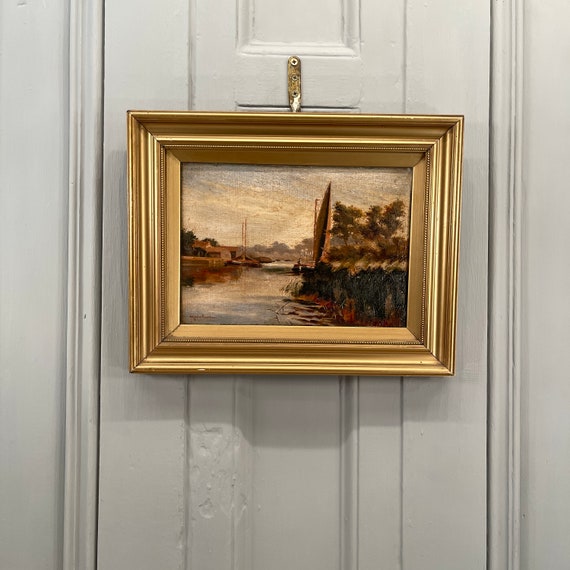This vertical rectangular photograph captures a painting hanging on a door. The door, closed and white, features wooden molding on both sides. The wall surrounding the door is also white. The painting, set in an ornate, multi-beveled gold frame, depicts a tranquil outdoor scene likely inspired by the 1800s or late 1700s pastoral style. Within the painting, a murky, brownish-gray body of water reflects the surroundings, with sailboats gliding on the surface. On the right side, a steep, muddy bank rises to gray and brown tones, topped with green grass and trees. To the left, a housing area with brown rooftops and green trees is visible. The sky transitions from gray at the top to yellow and tan near the horizon. The painting hangs by a silver thread, secured with gold screws, and beneath it, the door shows signs of wear, marred with dents possibly caused by a hammer.